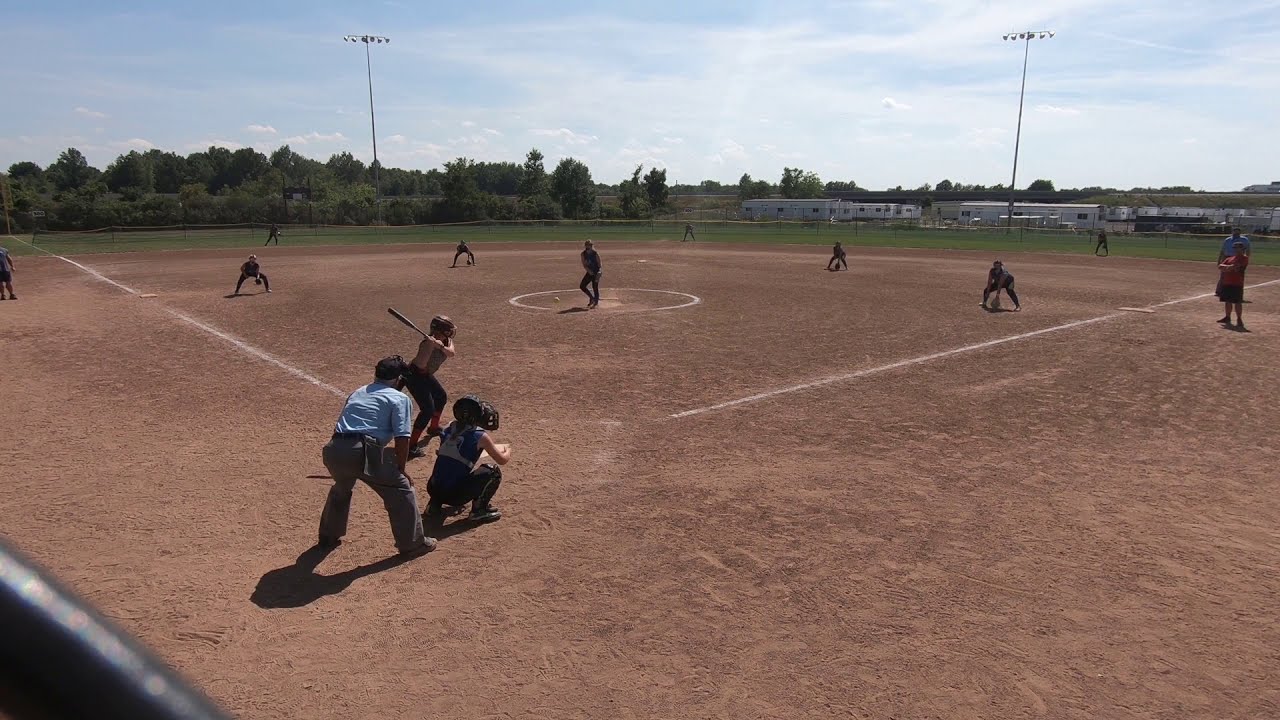This is a photorealistic image capturing an outdoor baseball game, focused from behind home plate. The players, likely young adolescents, are dressed casually in sweatpants and t-shirts rather than official uniforms. The ground consists of dark brown, sandy dirt marked with a white-drawn baseball diamond. Central to the image is the pitcher's mound, encircled by a white line. Ready to hit, a batter stands at home plate, donning a helmet, dark pants, and a brown shirt. An umpire, clad in a light blue shirt and black pants, stands behind the batter, with a catcher positioned further back in a blue shirt, gray pants, and a facemask. The infield and outfield players are spread out with their gloves ready on the ground. The infield is solely dirt, with sparse grass visible beyond the diamond. Surrounding the field is fencing, with more greenery and a few scattered trees to the left. Long, single-story white buildings, resembling trailers, line the right side. Tall lampposts tower over the field, ready to illuminate it at night, but for now, the bright blue sky with scattered white clouds indicates a sunny day.